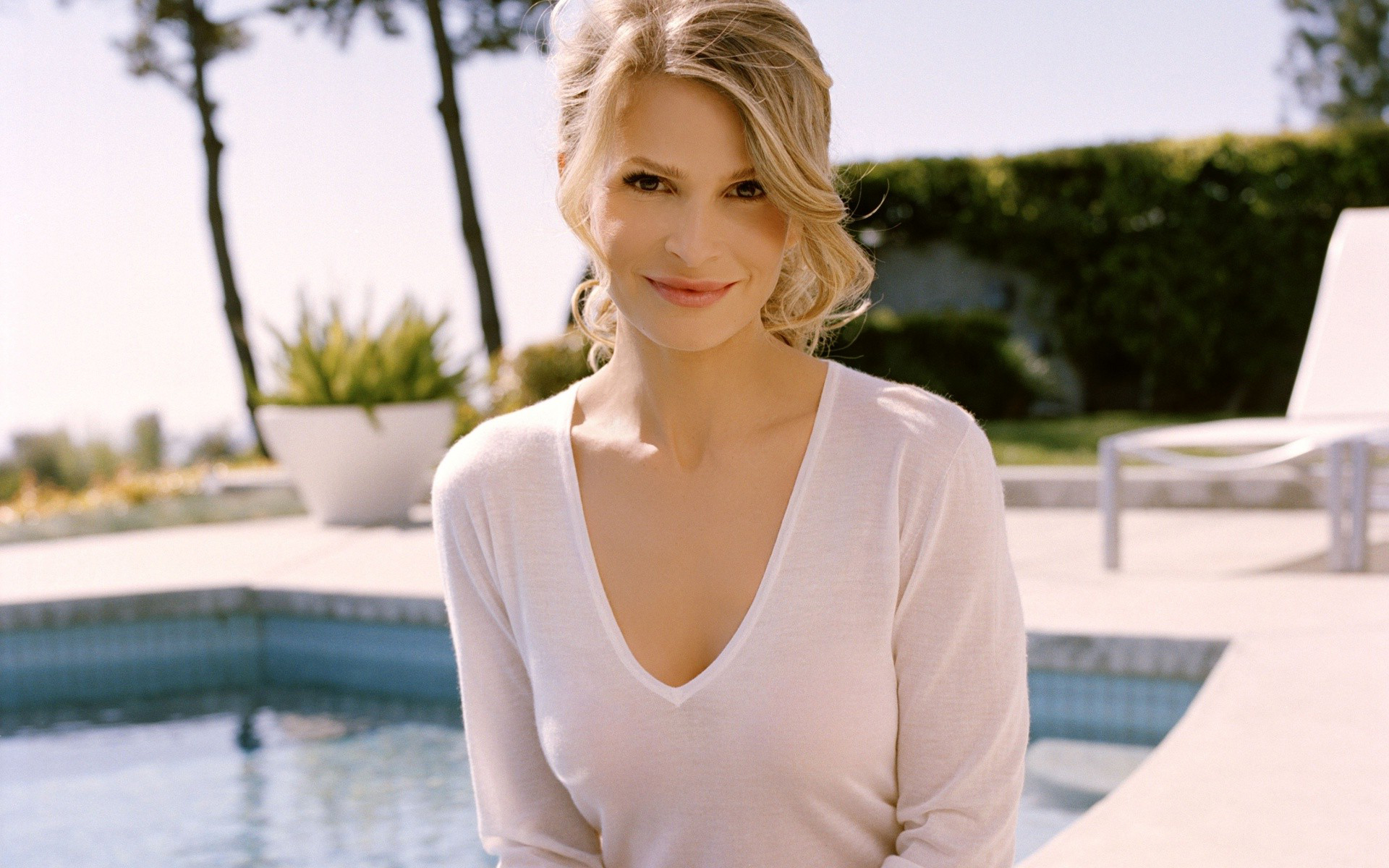The photo captures an outdoor scene featuring a serene pool deck framed by a blurred skyline in the background. A hedge with tall trees slightly out of focus forms a natural boundary, enhancing the tranquil ambiance. The pool deck is crafted from concrete and surrounds an in-ground pool, showcasing small blue square tiles within and steps descending into the water at the right corner. A large white pot containing a plant and a white lounge chair are positioned around the pool, adding to the inviting setting.

At the center of the image is an attractive woman who appears to be in her mid-twenties, characterized by delicate facial features and an innocent, youthful look. She has light blonde hair that is somewhat tousled and partially pulled back. Her long-sleeve white shirt with a scoop neck reveals much of her bare torso, complementing her subtle, closed-lip smile. She gazes slightly towards the camera, exuding a gentle, serene presence amidst the scenic backdrop.